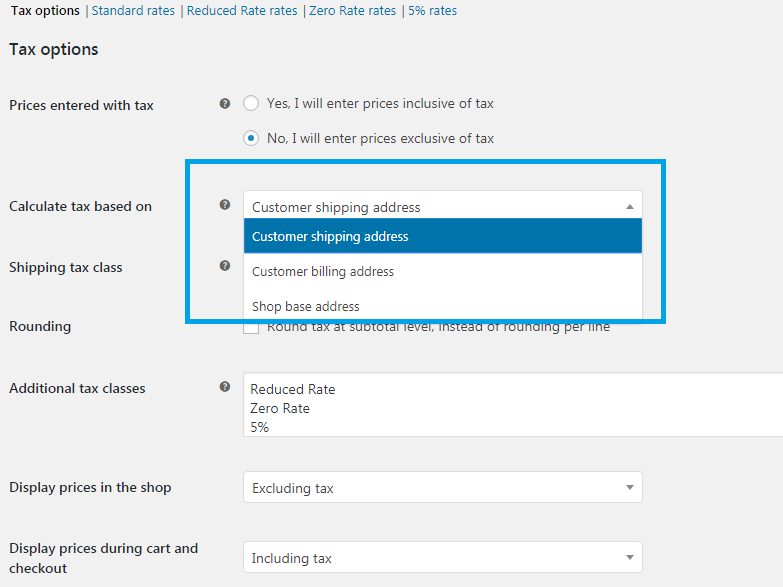The image depicts a screen capture of a desktop computer displaying an online application interface, specifically a page related to tax settings for an e-commerce platform. The upper left corner of the screen features a section labeled "Tax Options" in black text. Below this header, there are additional menu items listed in blue, which include "Standard Rates," "Reduced Rate Rates," "Zero Rate Rates," and "5% Rates."

On the left side of the screen, beneath the "Tax Options" heading, the same text "Tax Options" is repeated but in a larger font size. Below this larger heading, a series of options and configurations are listed in smaller print. These options include "Prices entered with tax," "Calculate tax based on shipping class," "Based on shipping tax class," "Rounding," and "Additional tax classes." Further options include "Display prices in the shop" and "Display prices during cart and checkout."

To the right side of the screen, various interactive elements are visible, such as radio buttons, dropdown menus, and text boxes. These elements likely correspond to the different tax settings and configurations that can be adjusted within the application. The design and layout suggest a detailed and user-configurable tax management system, aimed at facilitating the accurate calculation and display of taxes within an online shopping environment.